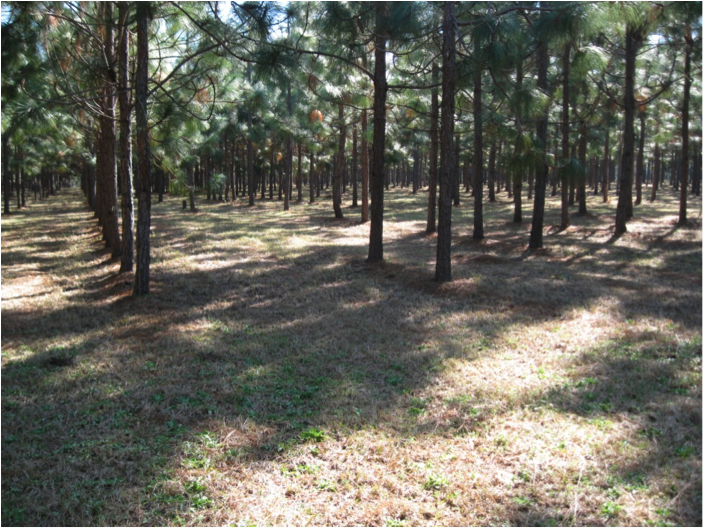The image is a color photograph depicting a dense forest or tree farm with tall conifer trees, likely pine, arranged in rows. The tops of the trees are not visible, focusing instead on the trunks and lower branches adorned with needle-shaped foliage. The ground is flat and sparsely covered with uneven patches of brown and green grass. Sunlight filters through the canopy, casting shadows across the landscape. Despite the regimented planting, some trees deviate from the orderly rows, adding a touch of natural irregularity. An old wooden fence runs across the foreground, enhancing the rustic charm of the scene. There are no people, animals, buildings, or mechanical objects visible in the photograph, leaving the viewer to appreciate the serene and structured beauty of the forest setting.